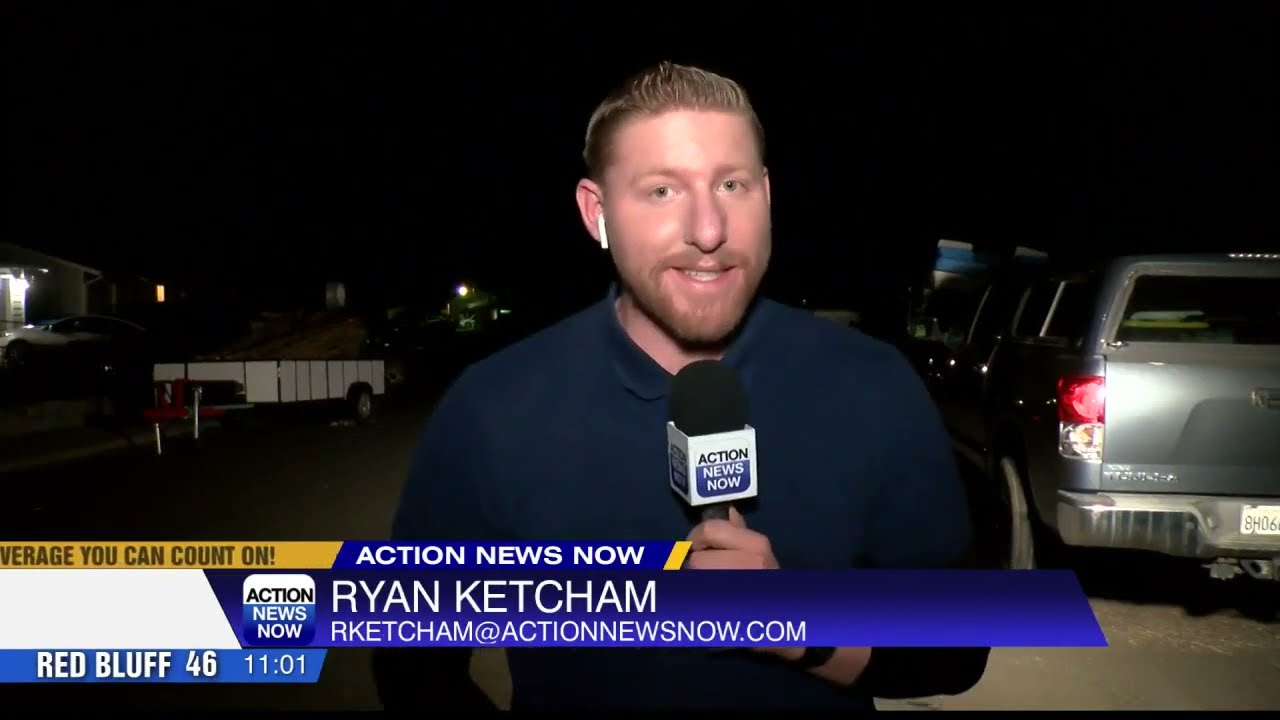In this detailed nighttime still frame from a news report, Ryan Ketcham, a Caucasian man in his late 20s with short light brown hair and a scruffy beard and mustache, stands in the middle of a street. He is the central figure in the image, wearing a long sleeve blue button-down shirt and holding a microphone in his left hand. The microphone's white square wrapper features the "Action News Now" logo, with dark blue lettering gradiating into a blue square with white lettering.

The setting is outdoors at night, as indicated by the dimly lit background, which is predominantly black, likely with either parked or moving cars around him. An Apple AirPod is visible in his right ear, suggesting he is receiving instructions or feedback during his reporting. The chyron across the bottom of the screen is divided into several parts: the top row featuring a gold section with the phrase "Coverage You Can Count On" in black lettering and a cobalt blue section with "Action News Now" in white lettering. The middle part of the chyron consists of a white bar with a diagonal edge that includes the "Action News Now" logo, followed by Ryan's name, "Ryan Ketcham," in white sans serif lettering over a gradient blue background. Below his name is his email, "RKetcham@ActionNewsNow.com." The lowest bar of the chyron is in a lighter blue, displaying the location "Red Bluff" along with the number "46" and the time "11:01" in narrow white lettering.